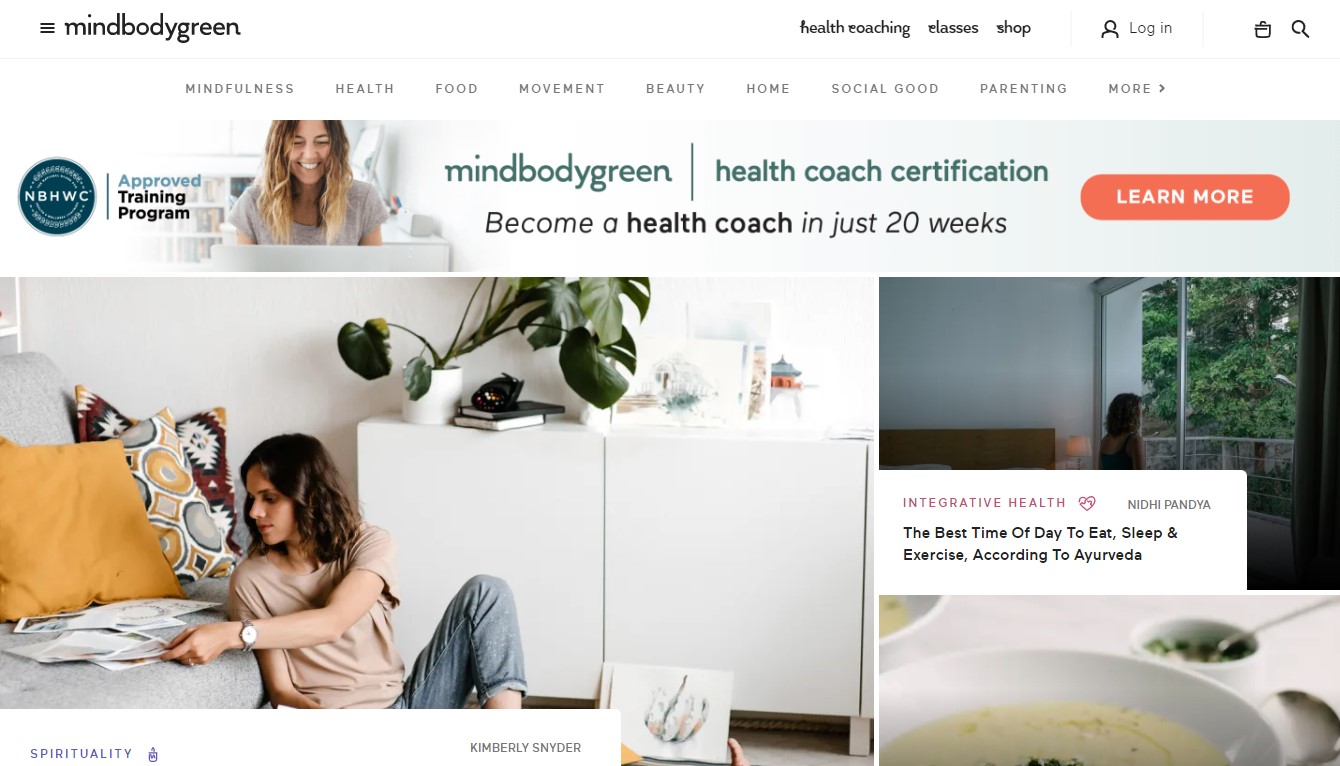The top left corner of the image features the Hamburger Magnus icon. Adjacent to it, a menu includes options such as mind, body, green, health, coaching, classes, shop, login, mindfulness, health, food, movement, beauty, home, social good, and parenting, along with a "more" button. The acronym VHWC is displayed next to a vertical line with the text "Approved Training Program."

Below, the text "Mind Body Green | Health Coach Certification" is prominently displayed. A caption reads, "Become a Health Coach in just 20 weeks," accompanied by a red oval button that invites viewers to "learn more."

In the background, the scene is predominantly white. To the left, there is a gray couch adorned with an orange pillow and some decorative shapes. A person wearing a pink shirt and blue jeans is sitting on the couch, leaning back and holding a paper. Nearby, white objects and plants are located on a counter.

On the right side of the image, text reads, "Integrative Health: The Best Time of Day to Eat, Sleep, and Exercise According to Your VEDA." Below this, a sink with a basin and liquid is visible. The backdrop includes a white wall with glass panels, beyond which green trees and pipes are seen, highlighted by reflective lighting.